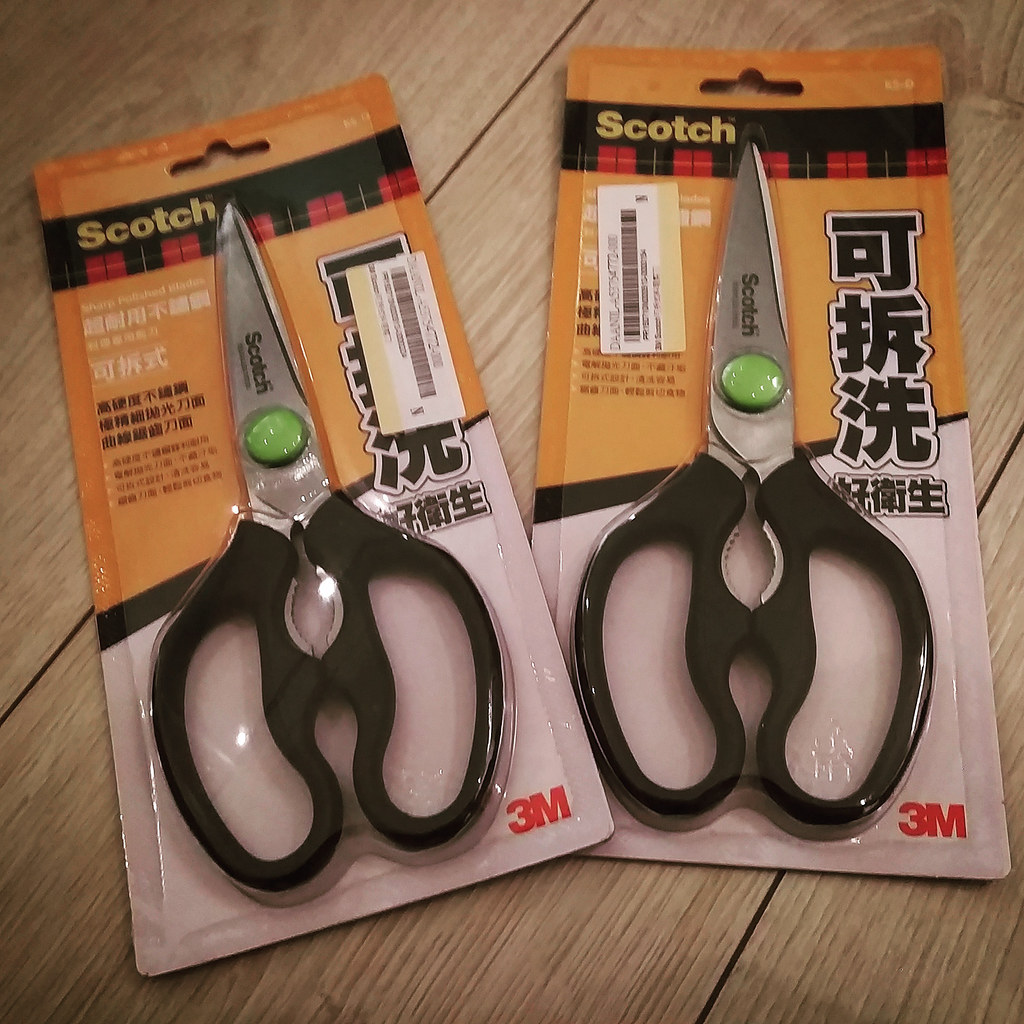The photograph features two identical packages of large shears, each with black handles and silver blades. The scissors, still sealed in brand-new plastic packaging, are displayed on a wooden table, the planks of which are clearly visible. Each pair of scissors has a distinctive green button at the joint where the blades pivot. The packaging prominently displays the brand name "Scotch" in large yellow letters against a black bar, positioned on a dark orange background with a lighter orange interior. A characteristic plaid pattern accompanies the branding at the top. Beneath the black bar, the packaging transitions to a white section at the bottom which includes a red "3M" logo in the bottom right corner. On the right side of the packaging, there are several sections of kanji text, suggesting the language might be Japanese. The package also features UPC sticker codes.